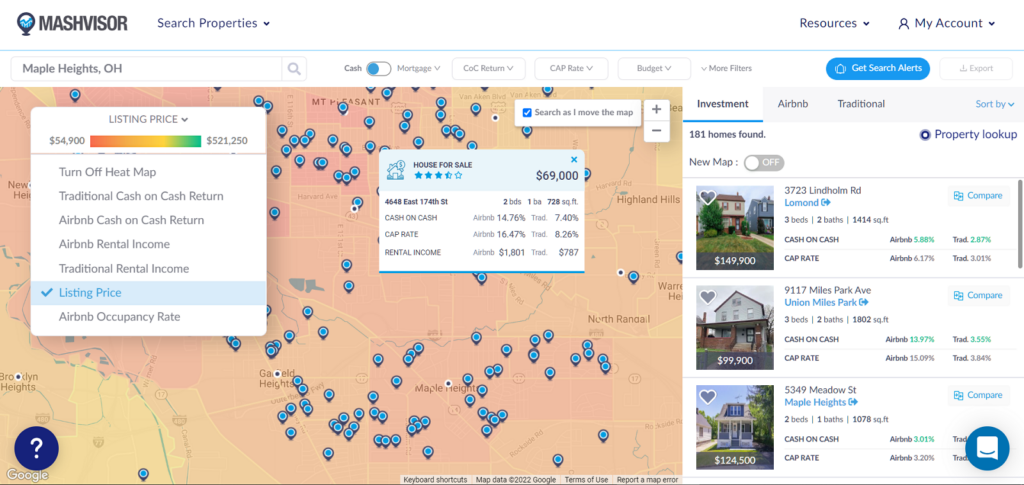Caption: 

A detailed screenshot of a property purchasing website, "MASH Pfizer," showcasing several housing listings in Maple Heights, Ohio. The central feature is a map cluttered with noted GPS locations signifying various listings, which are categorized by listing prices. The user interface also provides the option to toggle various heat maps for Traditional Cash on Cash Returns, Airbnb Cash on Cash Returns, Airbnb Rental Income, Traditional Rental Income, Listing Price, and Airbnb Occupancy Rate. On the right-hand side, there are three highlighted property listings: one priced at $149,900, another unusually low-priced at $999, and the third at $124,500. Additional tabs and features on the website include options to search more properties, access resources, and manage accounts using a drop-down menu, providing a comprehensive tool for house-seekers and investors.